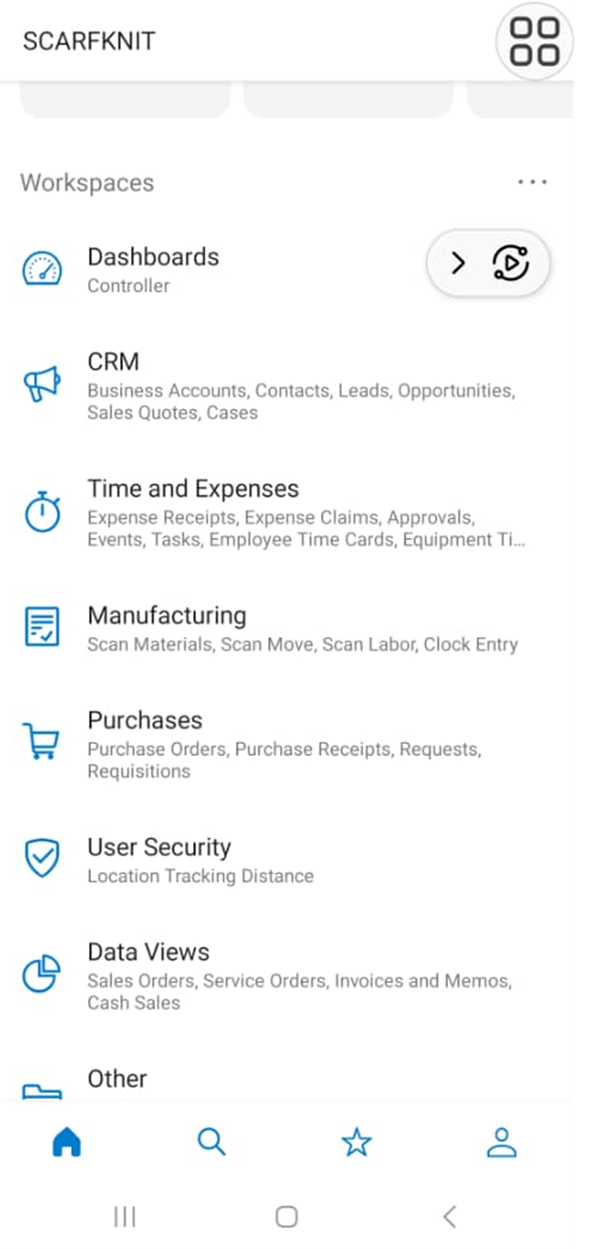The image appears to be a screenshot from a mobile application interface. At the top-left corner, the words "SCARF KNIT" are displayed in all capital letters. On the top-right, there is an icon resembling a circle divided into four quadrants or squares.

Below this section, partially obscured by the scrolling, are tabs with unreadable labels. Underneath these tabs, the word "Workspaces" is on the left, accompanied by a clickable three-dot menu on the right. 

Further down, there is an icon followed by the text "Dashboards Controller," and next to it is a button that resembles a play or repeat arrow. 

Below this, an icon that looks like a megaphone leads the section titled "CRM," which includes subsections for "Business Accounts," "Contacts," "Leads," "Opportunities," "Sales," "Quotes," and "Cases."

Next, an alarm clock icon introduces the "Time and Expenses" section, detailing "Expense Receipts," "Expense Claims," "Approvals," "Events," "Tasks," "Employee Time Cards," and "Equipment."

Following that is an icon of a piece of paper with a check mark, marking the "Manufacturing" section with options like "Scan Material," "Scan Move," "Scan Labor," and "Clock Entry."

A shopping cart icon highlights the "Purchases" section, including "Purchase Orders," "Purchase Receipts," "Requests," and "Requisitions."

Subsequently, a shield with a check mark signifies the "User Security" section, featuring "Location Tracking" and "Distance."

The next segment, introduced by a pie chart-like icon missing a triangle piece, is "Data Views," with entries for "Sales Orders," "Service Orders," "Invoices and Memos," and "Cash Sales."

Lastly, a split folder icon labels the "Other" section.

At the bottom of the screen are navigation buttons: a home icon, a search icon, a star icon, and a people icon.